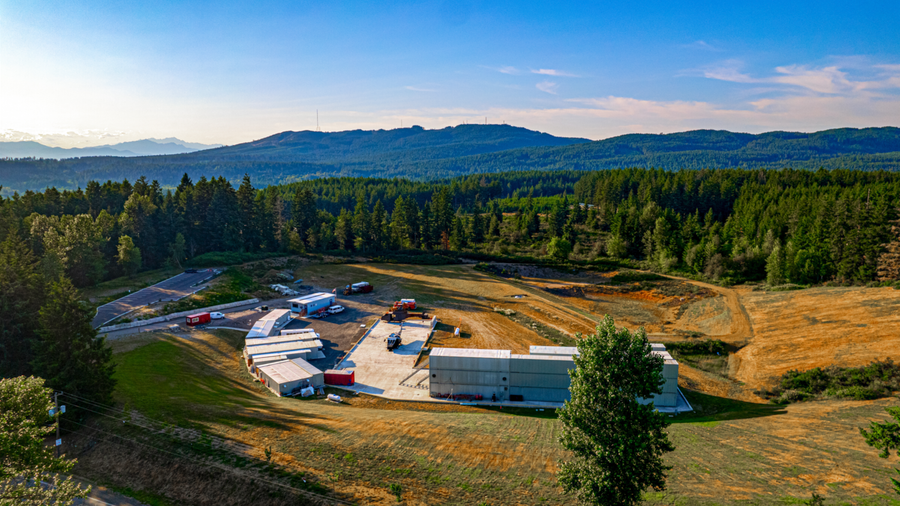This aerial photograph captures a vast, bucolic landscape dominated by lush, green forests and a sea of evergreen trees, primarily Douglas firs, that blanket the foreground and roll into the distant hills and mountains. The mountains themselves are draped with dense forest, creating a seamless stretch of natural beauty. The sky above is a vibrant blue, partially adorned with wispy clouds and a distinct pink hue to the right, hinting at either sunrise or sunset.

At the center of this verdant expanse lies a valley where industrial elements starkly contrast the surrounding natural splendor. Here, concrete structures, including a building and a parking lot with cars, punctuate the otherwise green terrain. A network of roads and dirt paths crisscrosses the open field, which seems to be an active construction site populated with trailers, vans, and trucks. Divots in the ground evidence ongoing work. The sunshine illuminates the scene, casting a bright light that further highlights the juxtaposition between peaceful nature and industrious human activity. Additionally, a large antenna is perched on one of the mountains, just left of the center, indicating possible communication infrastructure. This combination of untouched wilderness and human development creates a uniquely captivating and complex landscape.